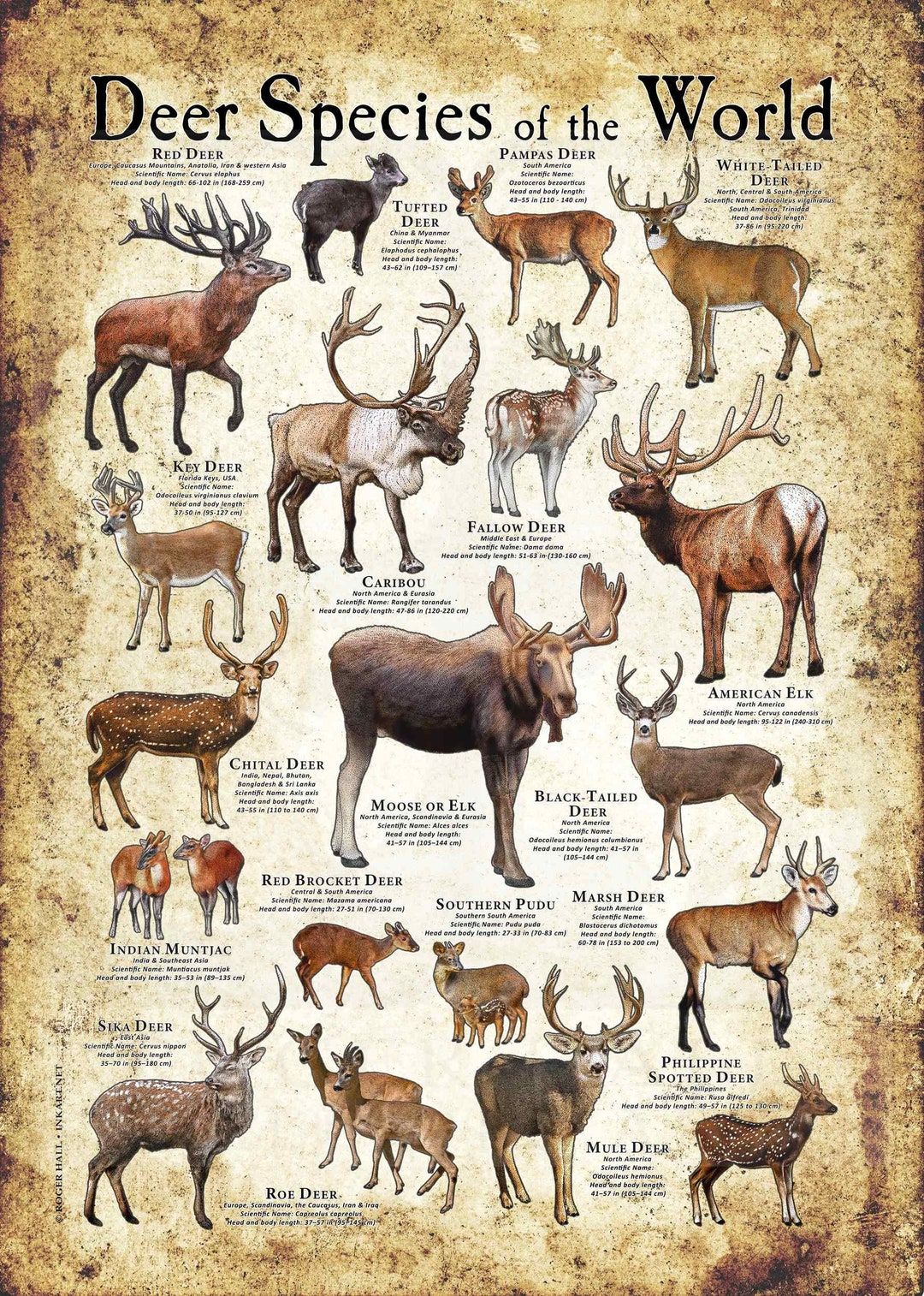The image is an infographic titled "Deer Species of the World," set on an old, damaged, and brown-colored piece of paper. The title is prominently displayed at the top in black text. The infographic features various colored illustrations of different deer species, each accompanied by a small descriptive paragraph. Species included are the Red Deer, Tufted Deer, Pampas Deer, White-tailed Deer, American Elk, Fallow Deer, Caribou, Key Deer, Chital Deer, Moose (or Elk), Red Brocket Deer, Indian Muntjac, Sika Deer, Roe Deer, Mule Deer, Philippine Spotted Deer, Marsh Deer, Black-tailed Deer, Southern Pudu, among others. The illustrations are detailed, showing differences in size, antler presence, and type: for instance, some deer have large or small antlers, while others have none. The aged appearance of the paper and extensive detailing of each species give the infographic a vintage and educational aesthetic.